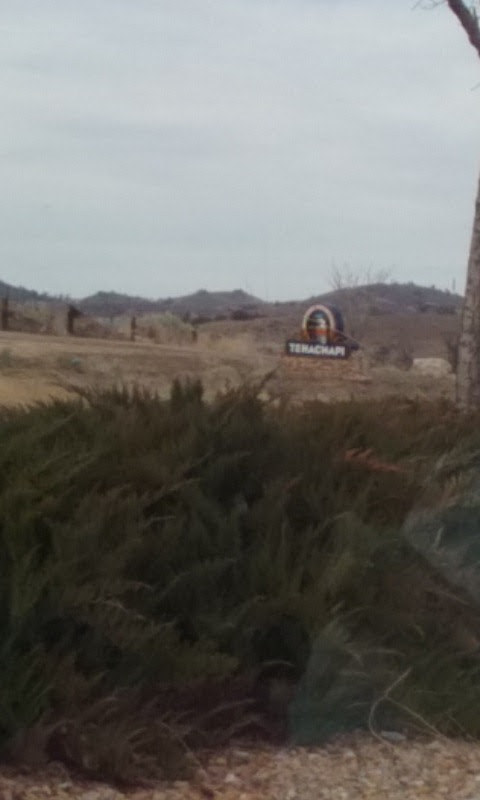This photograph captures an outdoor scene set in a desolate, arid landscape. The terrain is composed of rocky, sandy ground and dotted with scrubby evergreen shrubs and overgrown bushes in the foreground. Among the greenery, the dominant color is a dark, rich green. The landscape extends to a wide, open plain, and in the distance, you can make out several hills or low mountains under a partly cloudy, blue-gray sky, suggesting it might be a somewhat overcast day. A clear sign of human presence is visible in the background: a pair of signs, though they are blurry and difficult to read. One of the signs is circular with colorful elements, while the other is longer and bears the letters "T-E-H-A-C-H-A-P-I." The slightly out-of-focus quality of the photograph adds a layer of abstraction, making fine details hard to discern.